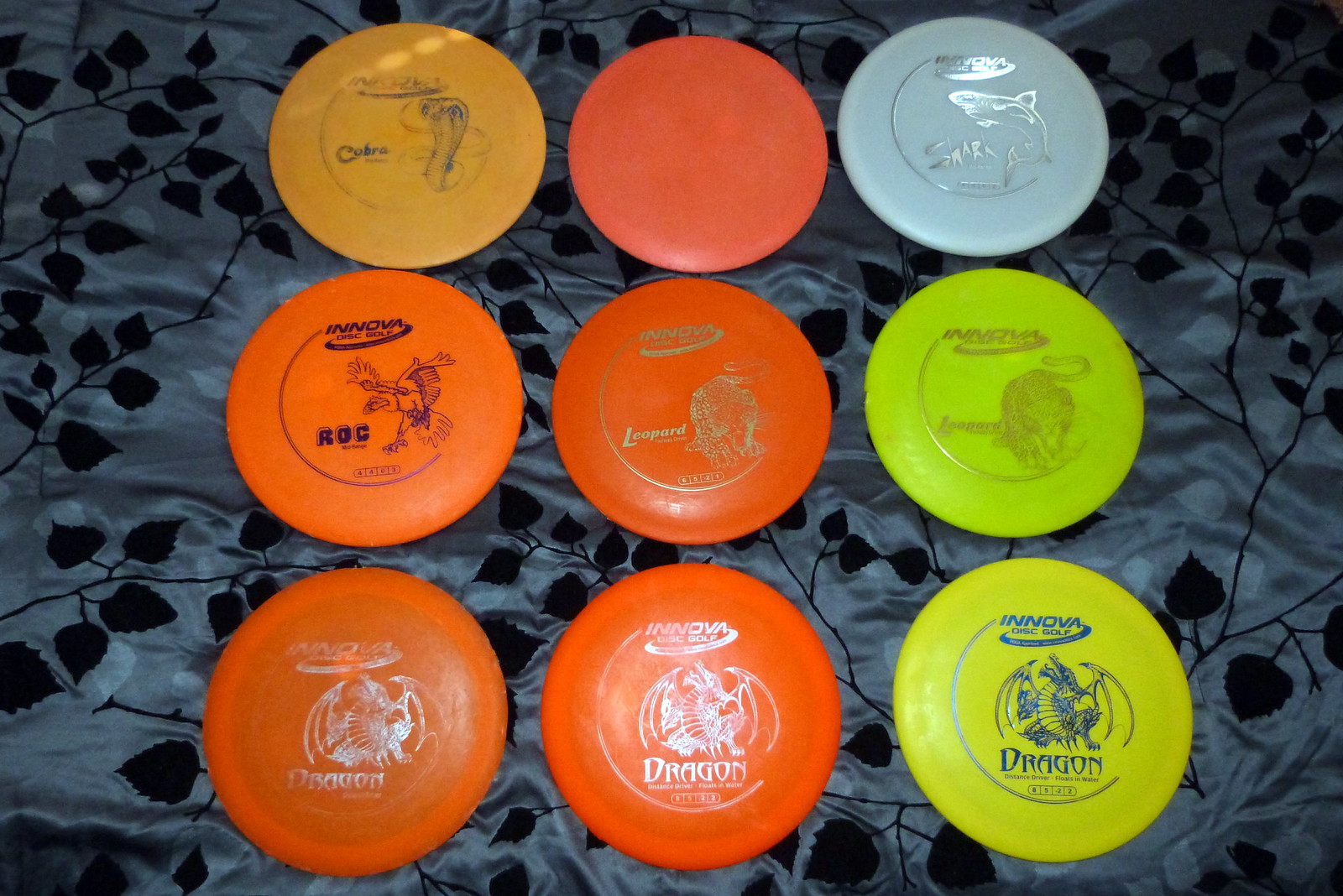The photograph showcases nine frisbees meticulously arranged in a 3x3 grid on a bluish fabric adorned with a black leaf-vine pattern. The frisbees, primarily in shades of reddish-orange, also include variations in lime green, blue, and yellow. Each frisbee features unique artwork and text, with some depicting animals such as cobras, sharks, dragons, leopards, and eagles, all marked with the brand "Innova Disc Golf." The mustard yellow frisbee displays a cobra, while the blue one features a shark. In the middle row, the frisbees include images of birds, whereas the bottom row comprises discs with dragon emblems. The fabric beneath the frisbees is slightly wrinkled, providing a casual, amateur backdrop to the vibrant display of frisbees.